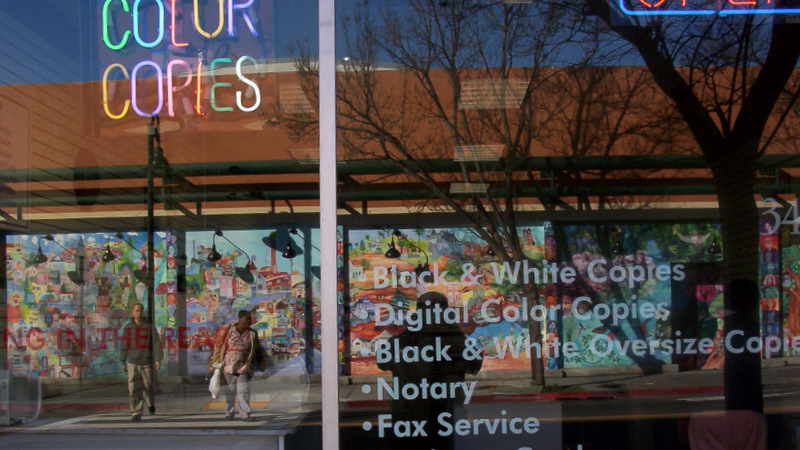This wide rectangular image captures the highly reflective window of a storefront, blending a vivid street scene with visible details inside the store. Reflections on the window reveal a brown building at the top and a green metal overpass spanning a gray sidewalk, all adding urban context to the image. On the left, two individuals are seen crossing a white crosswalk, while the silhouette of a leafless tree occupies the right side. Inside the store, in the top left corner, a rainbow-colored light sign brightly reads "color copies," with each letter a different hue of the rainbow. The store's services are listed in white font on the bottom right side of the window: "black and white copies," "digital color copies," "black and white oversized copies," "notary," and "fax service," vertically arranged to attract attention. This detailed setup effectively showcases both the lively urban environment outside and the business offerings inside.